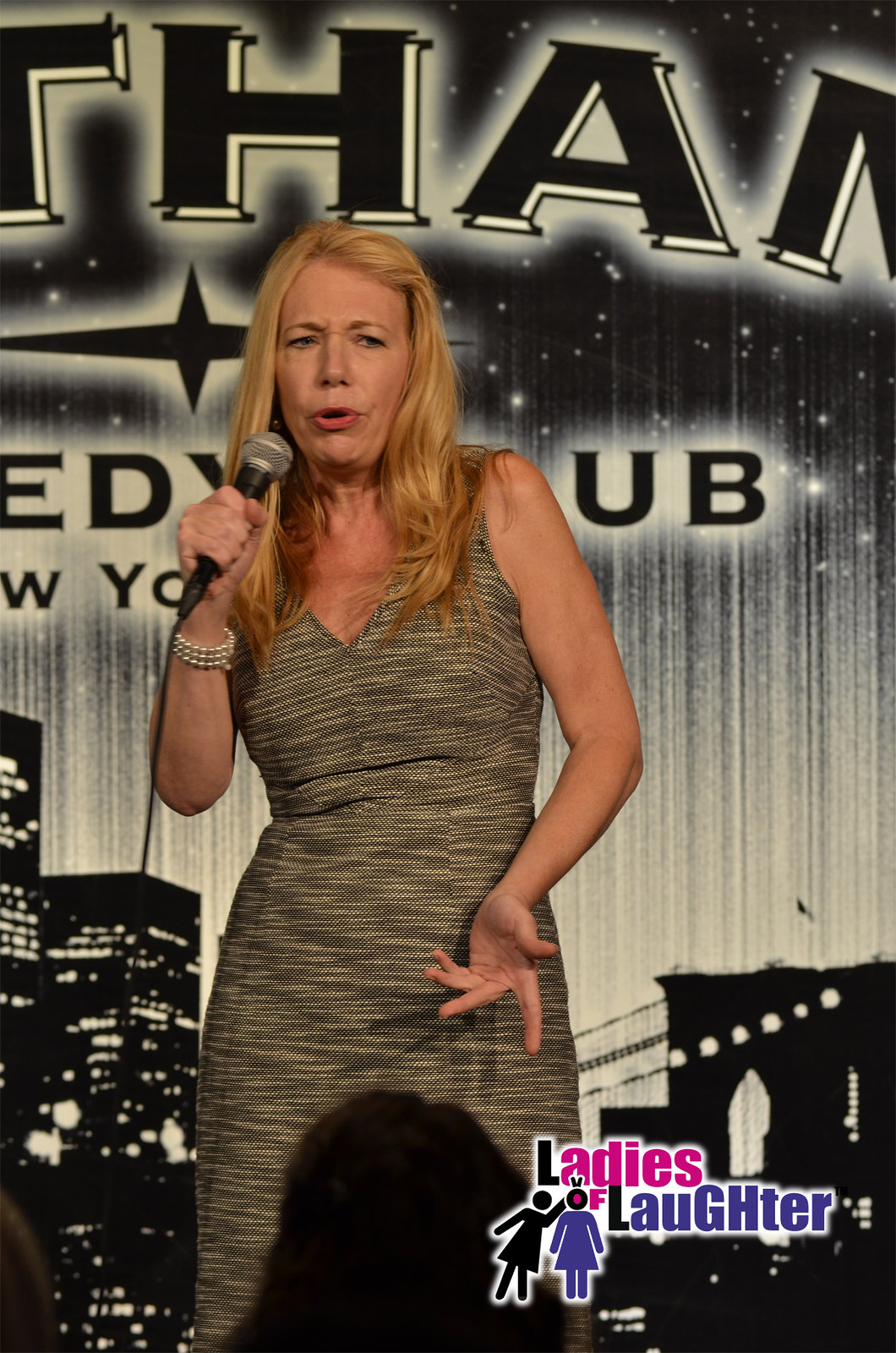The image is a color photograph in portrait orientation depicting a female comedian standing at the center, wearing a beige tweed halter dress and holding a microphone to her mouth with her right hand. Her long blonde hair cascades over her shoulders as her left hand is spread out in a gesture. She appears to be performing, likely telling jokes, to an audience whose heads are visible at the bottom of the image. The backdrop features partially visible text reading "Gotham Comedy Club New York" with certain letters obscured. The top part of the backdrop has large, bold white-bordered letters, and the bottom part includes a black silhouette of New York City buildings with white windows. In the right lower corner, a logo in pink and purple letters says "Ladies of Laughter" next to caricatures of two women. The setting appears to be indoors, possibly at a comedy club during nighttime, with a color palette that includes white, black, various shades of gray, pink, purple, tan, and a touch of brown.